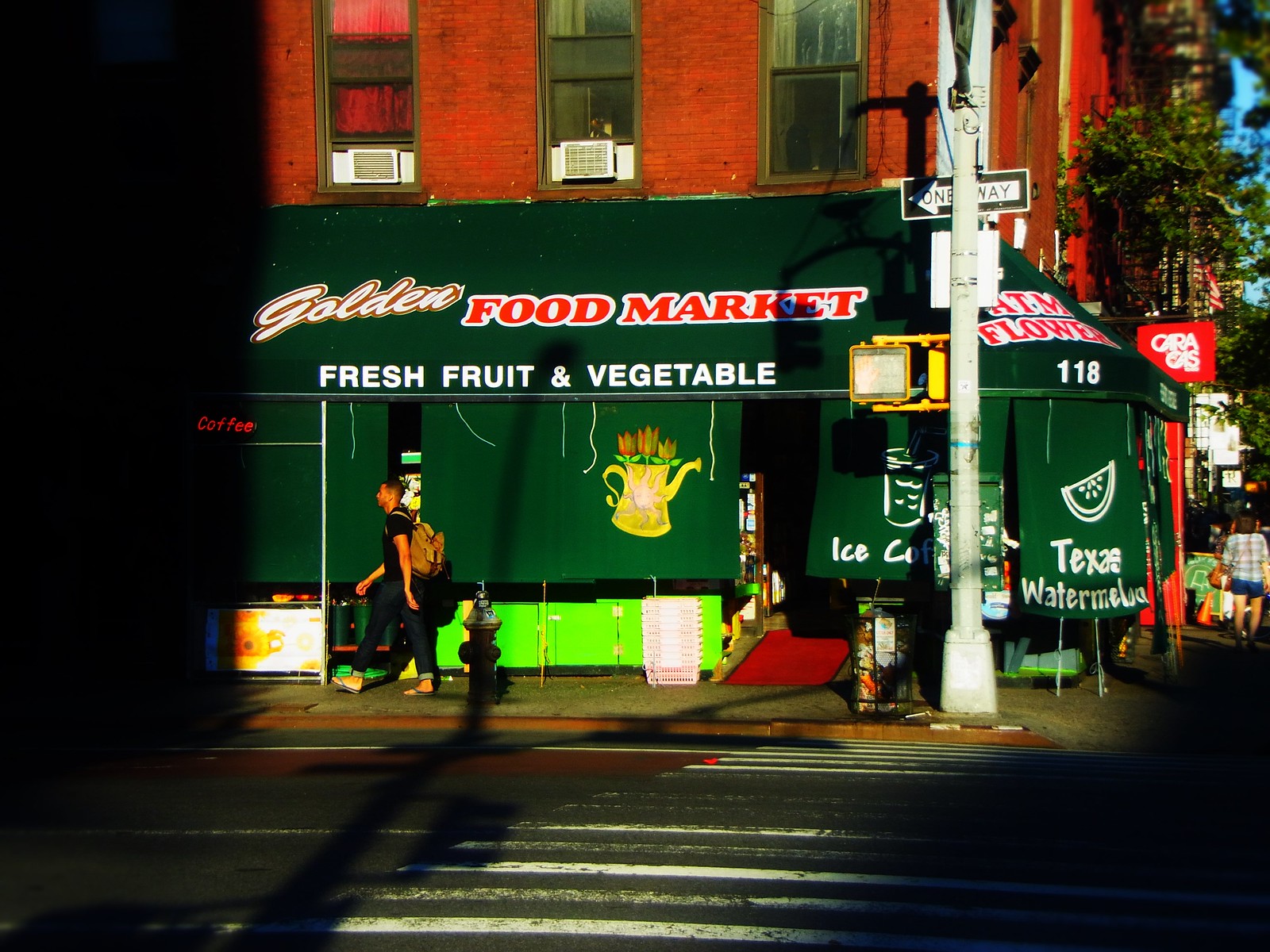The image captures an outdoor urban scene dominated by a large red brick building with three distinct windows—one with a red curtain and two with green curtains. In front of this building, there is a short green-sided building with the sign "GOLDEN FOOD MARKET" in bold letters. Below the main sign, in white letters, it reads "FRESH FRUIT & VEGETABLE," accompanied by an illustration of a yellow watering can with red flowers. Near the building, there are promotional signs for "TEXAS WATERMELON" and "ICE COFFEE." A white street post with a one-way sign pointing left stands prominently in front, and a few pedestrians, including a man in a dark shirt and pants with a brown backpack, are walking by. The scene is well-lit, indicating a bright midday with noticeable shadows. The foreground shows a segment of the street marked with white lines, enhancing the urban setting.